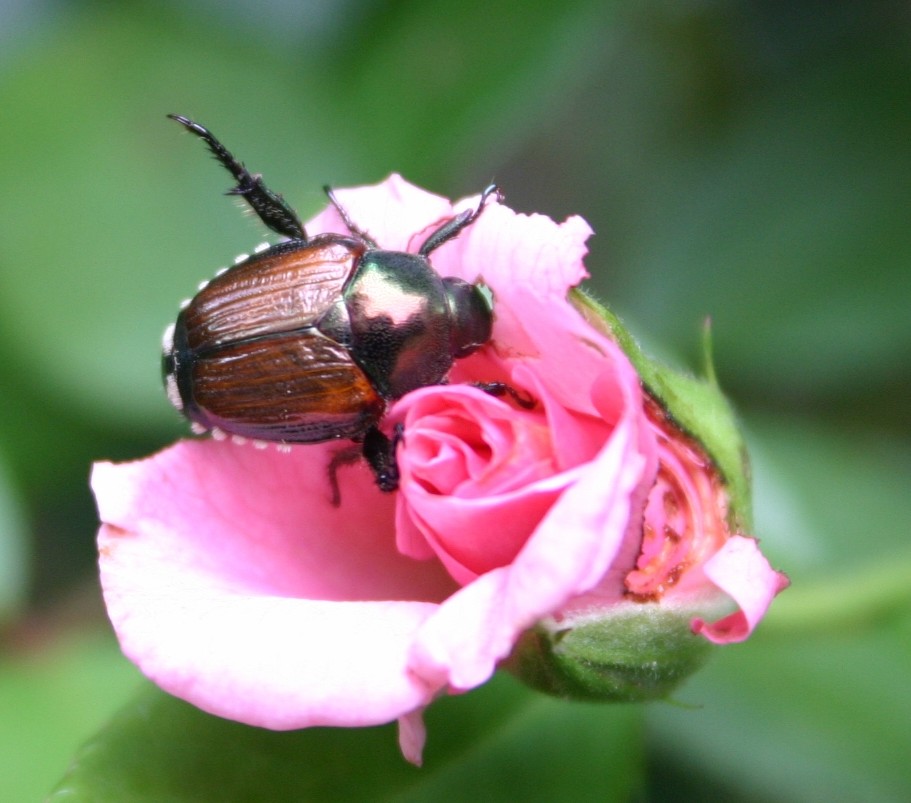The photograph captures a close-up of a beetle crawling on a partially bloomed, vibrantly pink rose. The beetle, facing the three o'clock position, features a black, reflective head and upper back that shimmers with hints of brown and green, reminiscent of an oil slick. Its legs are black and splayed out, while its wing covers exhibit a coppery-brown hue adorned with white dashes around the lower perimeter. The flower itself is surrounded by green foliage that is heavily blurred, emphasizing its vibrant pink petals as the focal point. The background features indistinct green tones, suggesting leaves and a stem. The beetle appears to be exploring the flower, possibly in search of food, amidst this vividly hued natural scene.